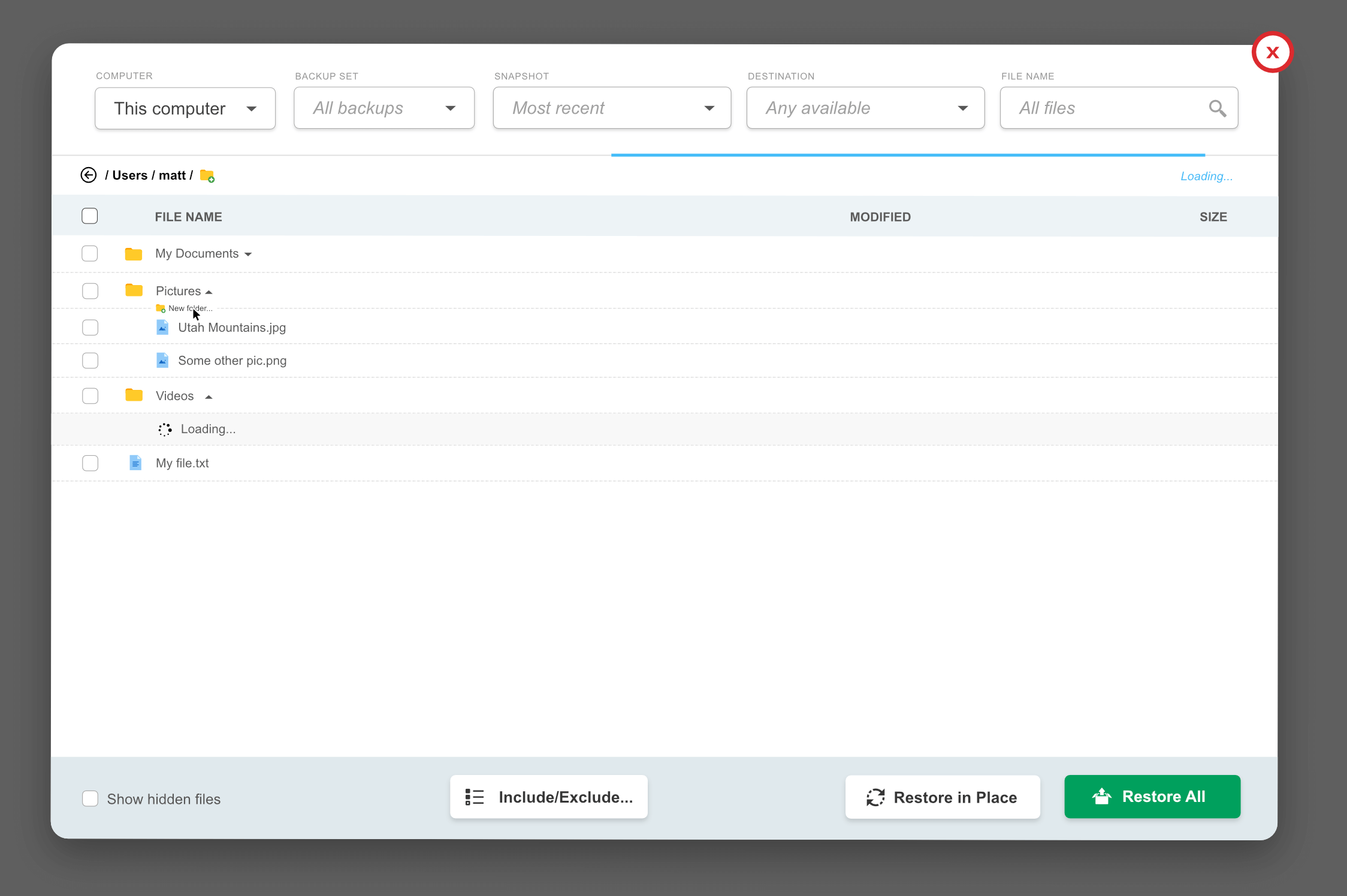This image displays a screenshot of a computer file management interface. At the top, there are several dropdown menus labeled "This Computer," "All Backups," "Most Recent," and "Occupation." Each of these dropdowns allows for specific selections. Next to these dropdowns is a search bar with a magnifying glass icon. 

Below the search bar, there are columns labeled "Users," with a folder icon nearby, "Modified," and "Size." Under these headers are several unchecked white checkboxes. The first checkbox is labeled "File Name." The second checkbox, also unchecked, is labeled "VY Documents" and is accompanied by a yellow folder icon. Similarly, another unchecked checkbox labeled "Pictures" is also shown with a yellow folder icon. There are smaller, less readable subfolders beneath "Pictures," one of which is labeled "Video" with yet another unchecked checkbox and yellow folder icon.

Further down, there is a section labeled "Loading" with a refresh button adjacent to it. At the bottom of the interface, options are displayed for managing files, which include buttons for "Show Hidden Files," "Include," "Exclude," "Restore in Place," and "Restore All." The overall interface presents a detailed overview of file management options and statuses.